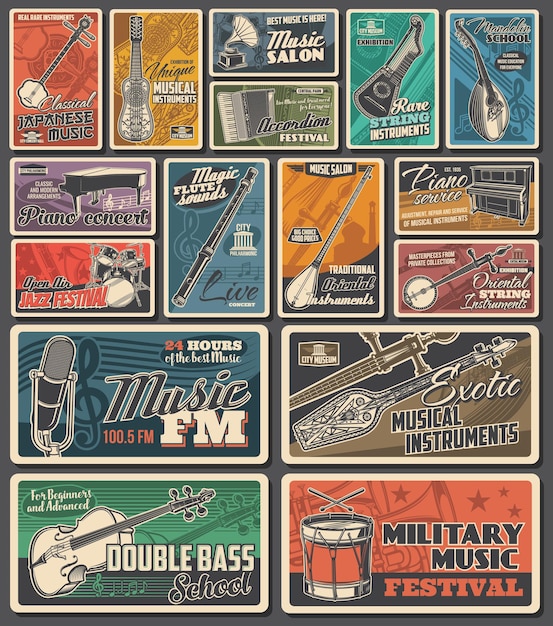The image appears to be an advertisement page characterized by its multicolored, cartoonish look, featuring a variety of rectangular banners, each dedicated to different music-related themes. Among these vibrant and creatively designed spots, notable ones include a banner for a "Military Music Festival," highlighted by a red drum graphic; another promoting a "Double Bass School," suitable for both beginners and advanced students, represented by a violin; and a section advertising "Music FM 100.5 FM," promising 24 hours of the best music with a small microphone illustration. Additional panels present themes like "Classical Japanese Music," "Exotic Musical Instruments," "Open-Air Jazz Festival," "Piano Concert," "Magic Flute Sounds," and "Oriental Instruments." Further down, there are mentions of piano services, rare string instruments, music salons, and an accordion festival, showcasing a rich tapestry of musical genres and instruments.